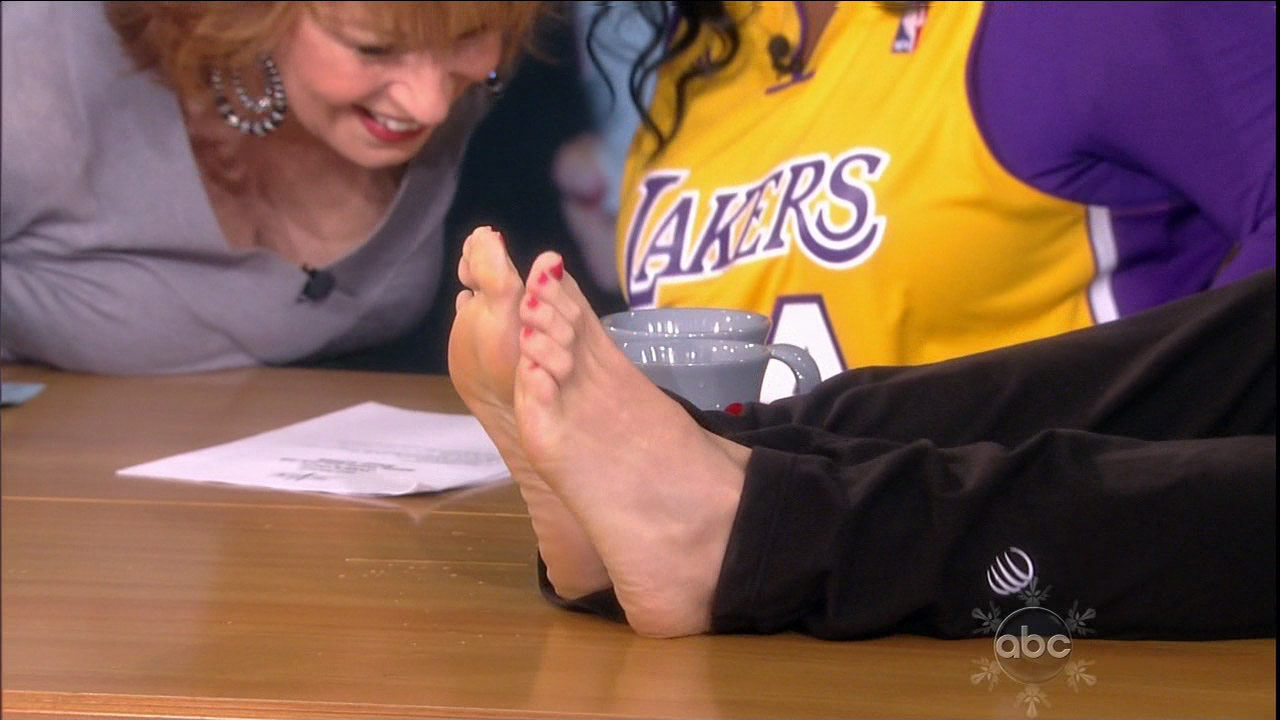In the photograph, a fun event is taking place centered around a table. A person, identifiable by their red-painted toenails as a female, is lying down or sitting with her legs straight on the table, wearing black pants. Her feet, adorned with red nail polish, are prominently featured. The brown table also holds some text-filled papers and two shiny gray porcelain cups, adding to the scene.

On the left side of the table, a smiling woman with blonde hair and earrings bends down to look at the feet. She is dressed in a gray outfit and has a microphone attached to her dress, suggesting she might be a presenter. Next to her, on the right side, stands another woman wearing a yellow and purple Lakers jersey. Though her face is not visible, part of her hair and a mic clipped to her outfit can be seen. In the bottom right corner of the image, near the lady's leg on the table, the ABC logo is displayed, likely as a watermark.